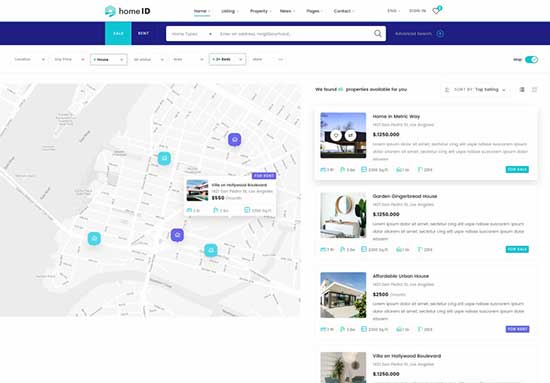This image is a screenshot from a webpage belonging to Home ID. At the top of the page, a Home ID logo is prominently displayed. The title bar, which appears to be a very dark blue or perhaps a deep purple, contains a search bar embedded within it. 

Central to the image is a map showcasing streets and various residential properties available for purchase or rent. Notably, the properties are color-coded: three properties are marked in teal, while two are marked in purple. A property has been selected or hovered over, indicated by a pop-up box displaying detailed information about that specific listing. 

On the far right side of the image, there is a list of four thumbnail images of different residences. Each listing is accompanied by a colored banner—two listings have a green teal banner, and one listing is marked with a purple banner. This detailed layout provides a clear visual representation of available properties and their statuses, enhancing the user’s ability to browse and select potential homes efficiently.